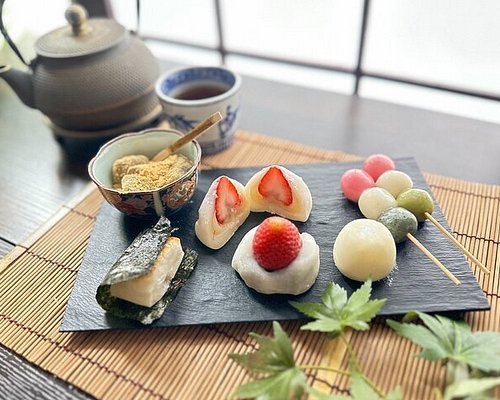In this striking indoor daytime photograph, a meticulously staged scene captures an array of culinary delights against a backdrop of natural light streaming through a white, vertically paneled window. The square image, devoid of text, showcases a black, wood-textured plate adorned with a variety of exquisite foods. In the lower left corner, a piece of sushi wrapped in seaweed nestles delicately next to a pastry garnished with a whole strawberry, while another pastry is sliced open to reveal the strawberry halves within. Centrally placed is a spherical, dough-like white mochi, flanked on the right by two skewers that alternate green, white, and pink spherical treats. The upper left corner of the plate features a cloisonné bowl containing cereal-like brown bits, with a spoon resting inside. Nearby, an iron-gray teapot and a ceramic cup of tea rest on a dark brown wooden table, partially covered by a bamboo placemat. In the bottom right corner, a dash of vivid green maple leaves adds a touch of natural beauty to this artful representation of traditional Japanese fare.